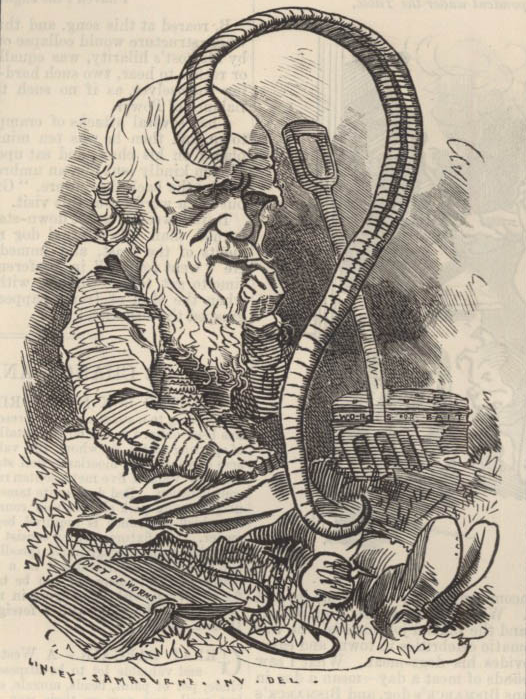The image depicts a detailed, hand-drawn, black-and-white cartoon of an older man with a long white beard and a bald head, sitting contemplatively on grass. His right finger is raised to his lips, suggesting deep thought or concern. The man, with exaggerated larger head proportions compared to his body, is dressed in a long shirt with a collar and boots. Surrounding him are several intricate objects: a pitchfork with its handle pointing upwards placed to his left, an open book on the ground to his right titled "Diet of Worms," and a large snake-like figure with its head hovering above him. The drawing, likely done with pencil or pen, showcases the man's pensive expression amidst a sparse background of creamy white paper, creating a striking focus on the central character and his surroundings.